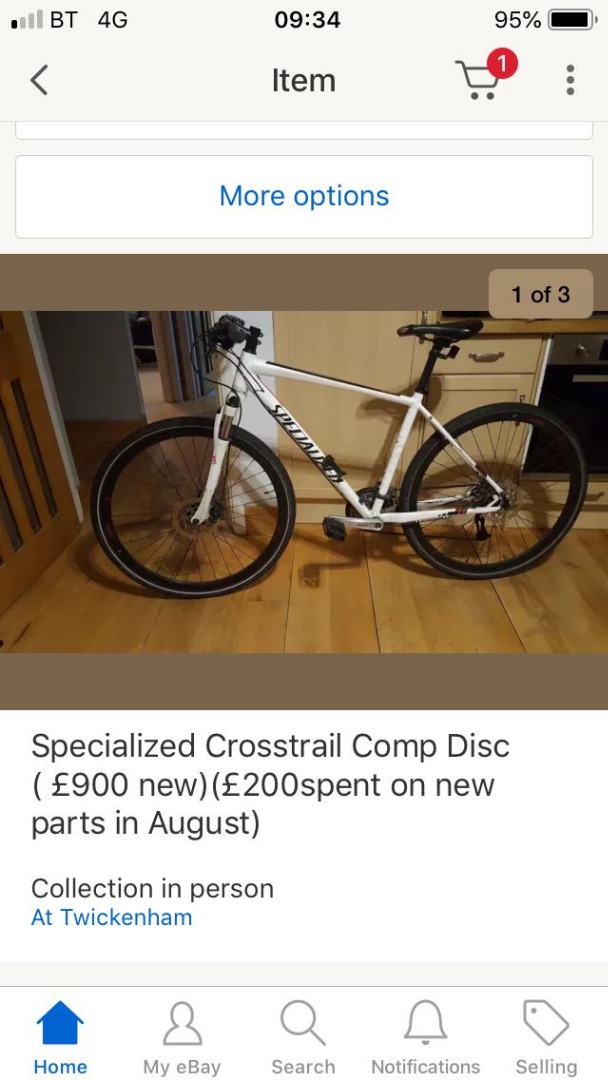This is a detailed screenshot of an eBay listing page. At the top, it features a header with the label "Item" and a back arrow icon to the left. To the right of the header, there is a red card icon and a vertical three dots icon for additional options. Below this header, there's a white button with the text "More options" in blue. The main content of the screenshot showcases an image of a white bicycle situated in a hallway. In the upper right corner of the image, it indicates "1 of 3" to denote multiple images. Below the image, the text reads "Specialized Crosstail Comp Disc." Additional details include the information that the bicycle originally costs £900 and recently had £200 spent on new parts in August. The listing specifies "Collection in person" and notes the location as "Twickenham" in blue text. At the bottom, there is a navigation bar with five icons: Home, eBay, Search, Notifications, and Selling. The Home icon is highlighted in blue, indicating the current active tab.